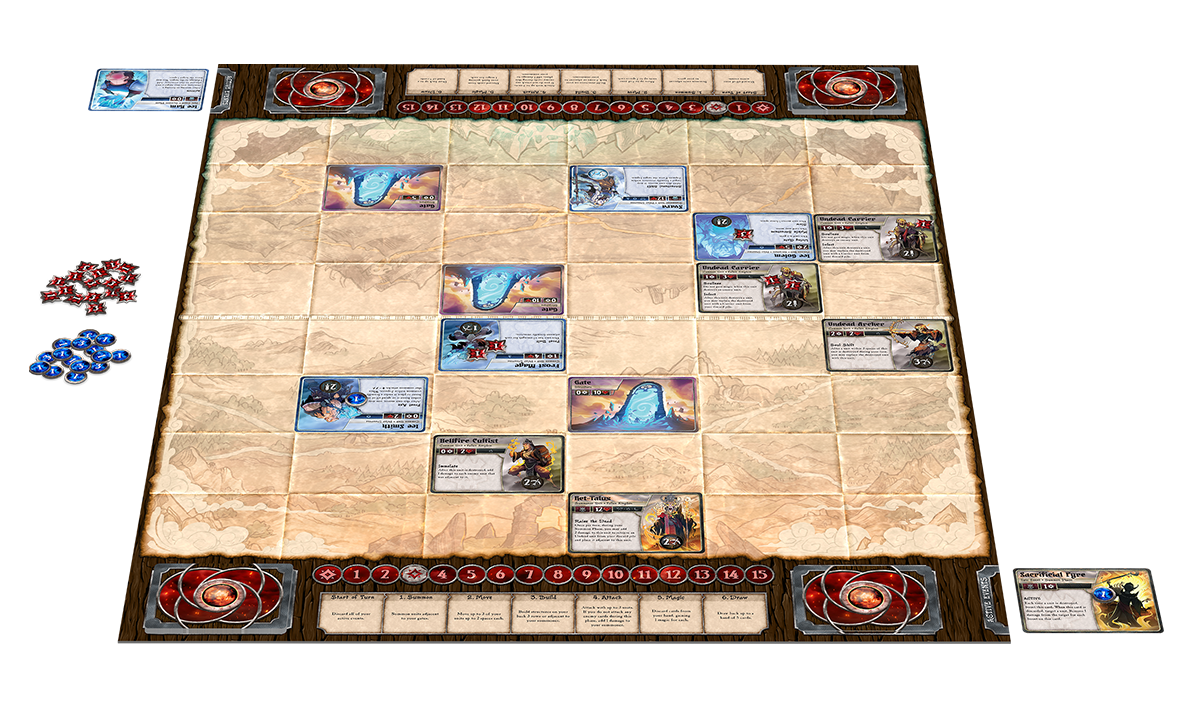The image shows a detailed game board from the board game "Summoner Wars." The board is an 8 by 6 grid of squares with a sand-colored map, darker in some areas and lightened spots suggesting water bodies. Despite the numerous blocks with writing, the text is illegible in this context. The board features cards positioned on twelve of the squares, with additional cards lying in the bottom right and upper left corners, hinting at gameplay elements. The board itself has a wooden bark-type background along its far and near sides, alongside a central dividing line. Each player's side features a row of numbers from 1-15, separated by star symbols and displayed within red circles. The setup appears to accommodate two players, with each side equipped with stacks resembling draw and discard piles. The exact mechanics of movement and further game details remain unclear without legible text, but the strategic placement of cards and the presence of chips colored in blue and red suggest complex gameplay elements.